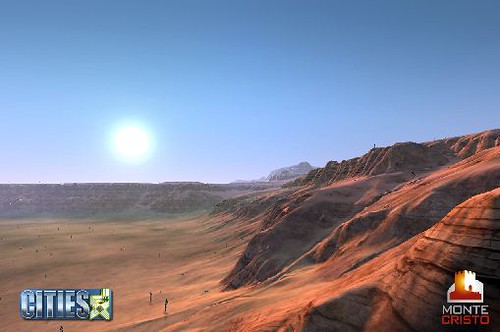The photograph appears to be part of an advertisement, characterized by a horizontal rectangle in the lower left corner that displays the word "CITIES" in bold blue capital letters. To the right of this text is an indistinct image. On the right side of the image, the name "Monte Cristo" is displayed, alongside a building logo in shades of white, red, and orange.

The image itself is stunning, featuring a flawlessly blue sky with a radiant white sun illuminating the scene. The horizon in the background is a soft gray. Prominent high mountains occupy the middle ground, transitioning seamlessly into lower plains. The foreground is dominated by pinkish sand, dotted with boulders that rise up and merge into flatter mountain surfaces. These geological features are painted in a subtle palette of grays, peaches, and pinks, creating a visually captivating landscape. Scattered throughout the scene are several small human figures, with one perched atop a mountain and others dispersed across the sandy terrain, resembling tiny dots. This intricate composition highlights the serene and sublime beauty of nature.